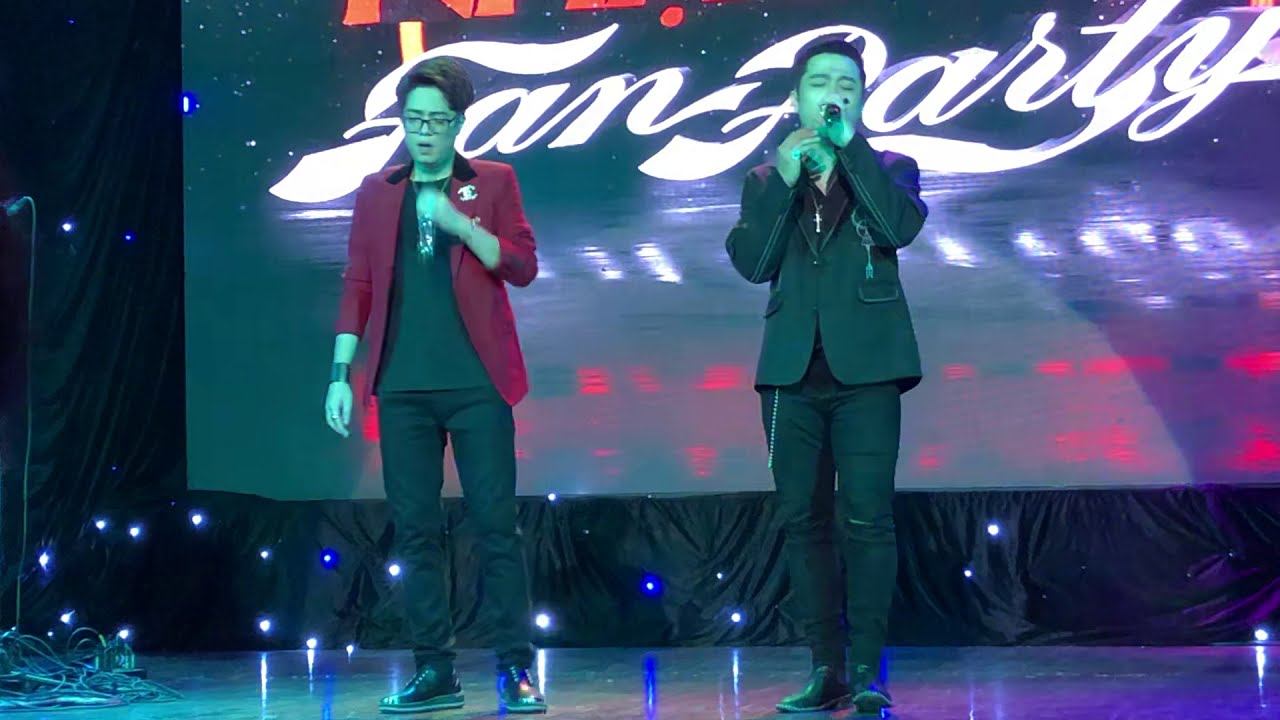The image captures a dynamic moment indoors featuring two young Asian male performers, likely in their early 20s, standing on a stage. The man on the left is dressed in a vibrant red jacket over a black shirt, black pants, and black shoes, accessorized with eyeglasses, a necklace, and holding a microphone in his left hand at chest level. The man on the right is clad in an all-black ensemble: a black jacket, black shirt, black pants, and black shoes, complemented by a cross necklace. Both performers have short, dark hair and their eyes closed, deeply immersed in their singing. The backdrop features a dark blue canvas with prominently displayed white script reading "Fan Party," surrounded by vibrant streaks of purple, red, and blue light. The stage floor is dotted with cords, adding to the authentic live performance setting, tinted with purplish-reddish hues from the stage lighting.